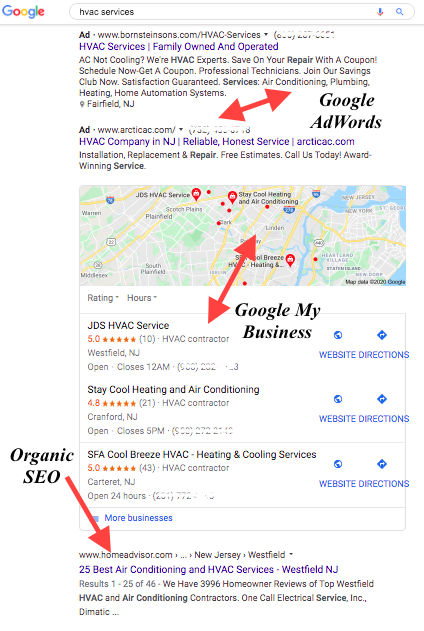This image displays a Google search results page for "HVAC services." At the top, there is a highlighted advertisement for Bernstein Sins, a family-owned and operated HVAC services provider. The ad highlights services for non-cooling HVAC systems and promotes savings on repairs with available coupons. The ad emphasizes professional technicians, satisfaction-guaranteed service, and expertise in air conditioning, plumbing, heating, and home automation systems. The company is located in Fairfield.

The second search result is for ANCTK.com, a reliable and honest HVAC service company based in New Jersey. This entry promises dependable service and links to an article on their website.

Between these two advertisements, there is a double red error message with black text that reads "quickly add weight." Below this, a map is displayed with another double red error pointing at it. The text under the map in black reads, "quickly my business." 

Further down, the image displays a listing for JTS HVAC Service with the tagline "Stay Cool Heating and Air Conditioning." Another listing, SFA Cool Breeze HVAC Heating and Cooling Services, appears just above a HomeAdvisor link. The HomeAdvisor entry lists the "25 Best Air Conditioning and HVAC Services in Westfield, NJ."

On the right side of the screen, there is another red error pointing to the HomeAdvisor entry with the text "organic SEO."